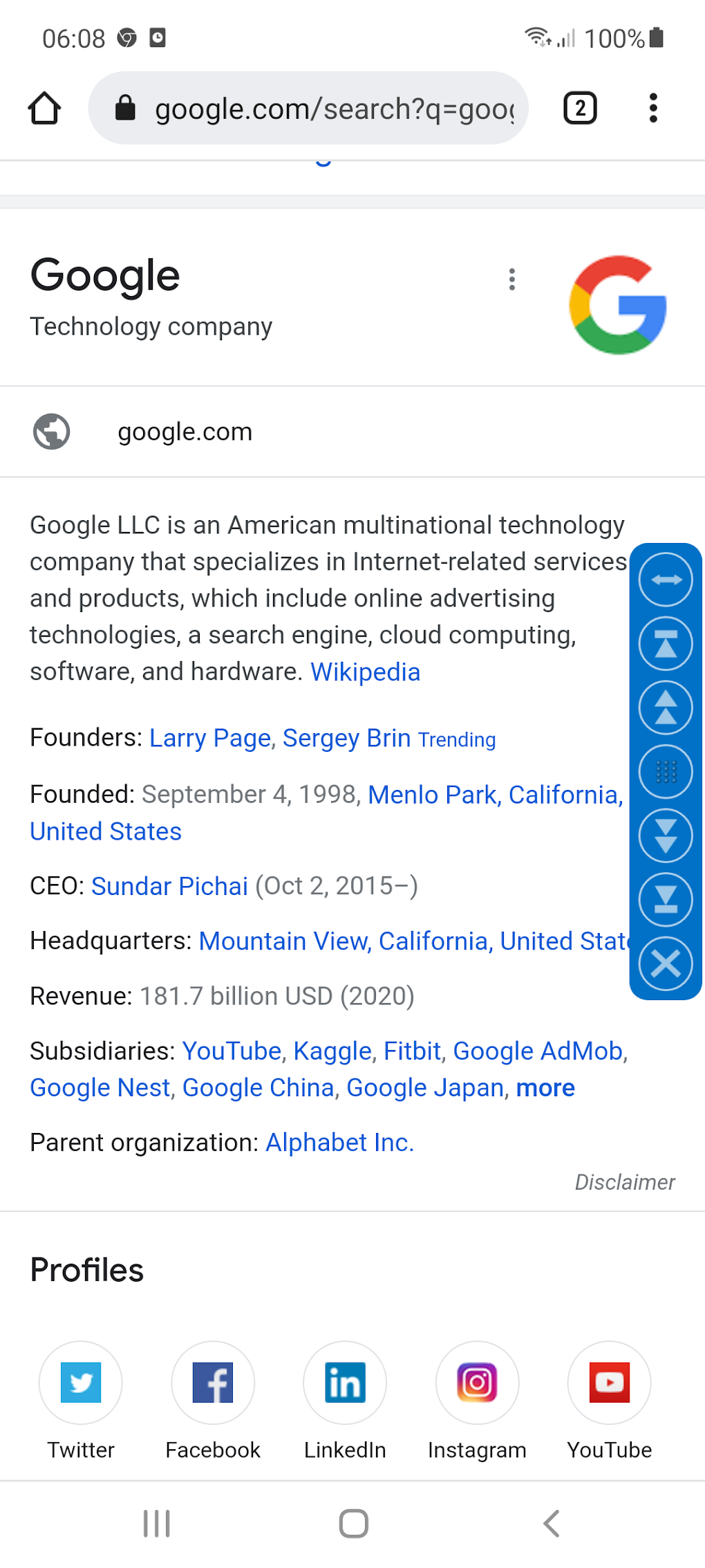A detailed screenshot of a smartphone's screen at the time of 6:08 AM or PM. The top status bar of the phone indicates that Wi-Fi is enabled with full signal strength, the mobile network has three bars of service, and the battery is fully charged at 100%. The screenshot was taken while the user was browsing the internet, specifically on a webpage accessed via Google Chrome.

At the very top of the browser, the homepage icon is visible beside a secure lock symbol indicating the URL "google.com" in the address bar. To the right, a small square with the number '2' indicates that two tabs are open. 

The content of the displayed tab is centered around Google, featuring the company's distinctive multi-colored 'G' logo in red, yellow, green, and blue. The webpage appears to be from Wikipedia, offering an overview of Google LLC. The description states that Google is an American multinational technology company that specializes in Internet-related services and products. This includes the realms of online advertising technologies, search engines, cloud computing, software, and hardware.

There's a world globe icon preceding "google.com" to emphasize its global presence. The page further lists details about the founders, Larry Page and Sergey Brin, as well as the company's inception date of September 4, 1998, in Menlo Park, California, USA. Additionally, the CEO is mentioned as Sundar Pichai along with a hyperlink presumably leading to further information on Wikipedia.